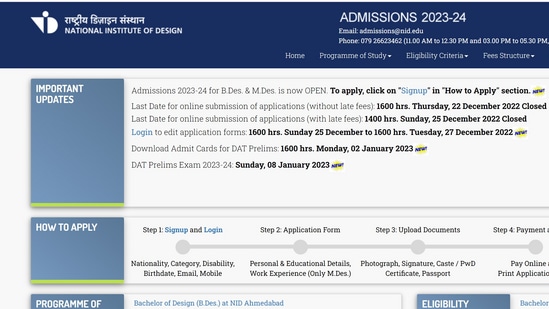Screen capture of the admissions web page for the National Institute of Design. At the top of the image, a dark blue horizontal bar spans across the frame. On the left side of this bar, the logo for the National Institute of Design is prominently displayed. On the right side, the text "Admissions 2023-2024" is written in white.

Below the dark blue bar, the page provides email and phone number information for inquiries. The main body of the image features important updates and instructions on how to apply. At the top of the "Important Updates" section, the text "Admissions 2023-2024 for BDES and MDES is now open. To apply click on sign up in the how to apply section" is highlighted in white.

This detailed information guides prospective students on how to initiate their application process for the Bachelor of Design (BDES) and Master of Design (MDES) programs for the 2023-2024 academic year.